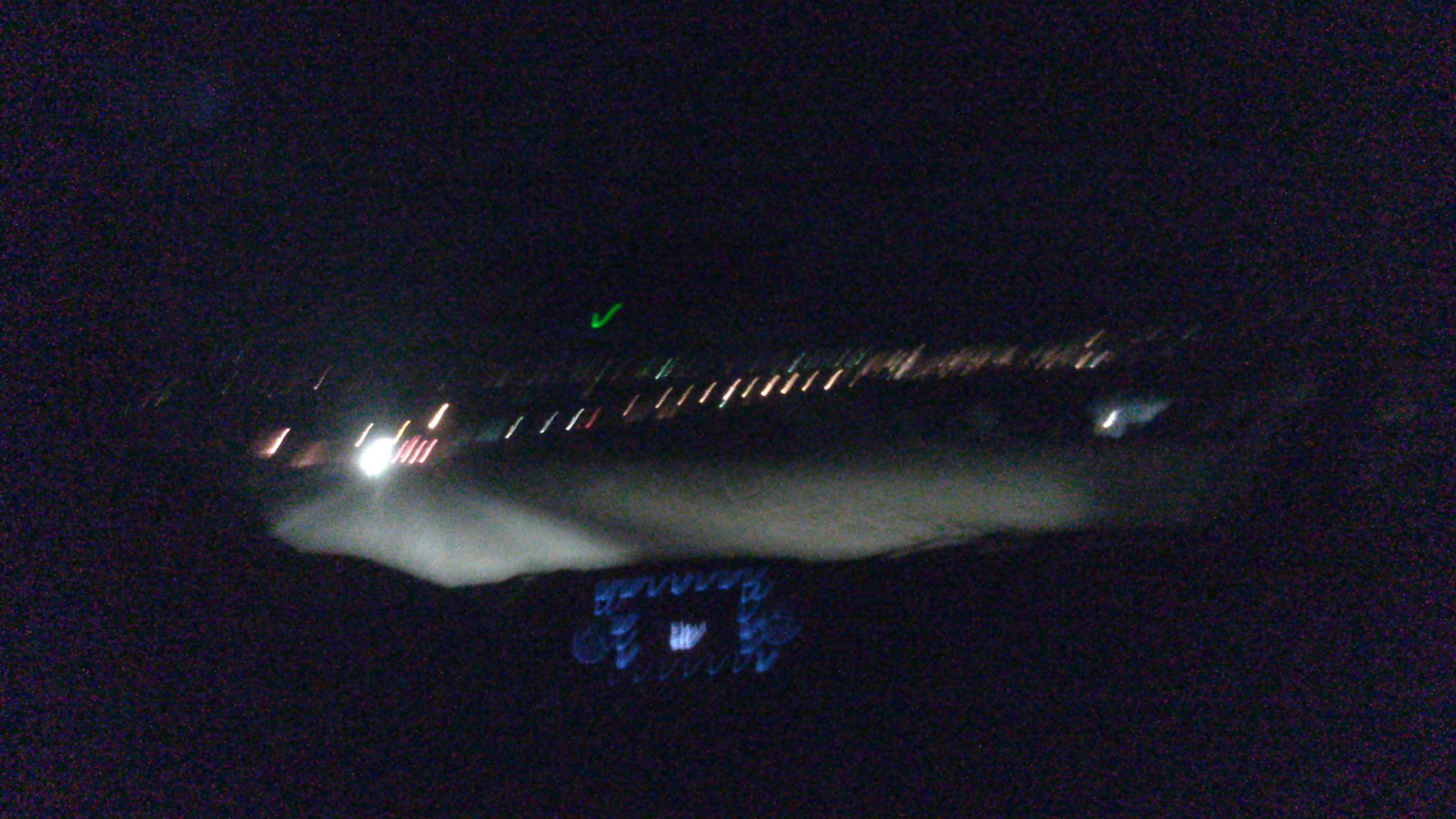A grainy and extremely blurry night-time photograph featuring an indistinct, large, tubular object dominating the center. A series of slit-like lights, mostly yellow with a few green ones, run horizontally across the image. A bright white light is distinctly visible near the left center within this row. Below the tubular object lies a pattern of blue rectangular dots, with one of the bottom row's rectangular lines dimly lit. Vaguely, white objects resembling bowling pins can be discerned in the center. The scene might depict an aircraft body landing, flying, or something entirely different.